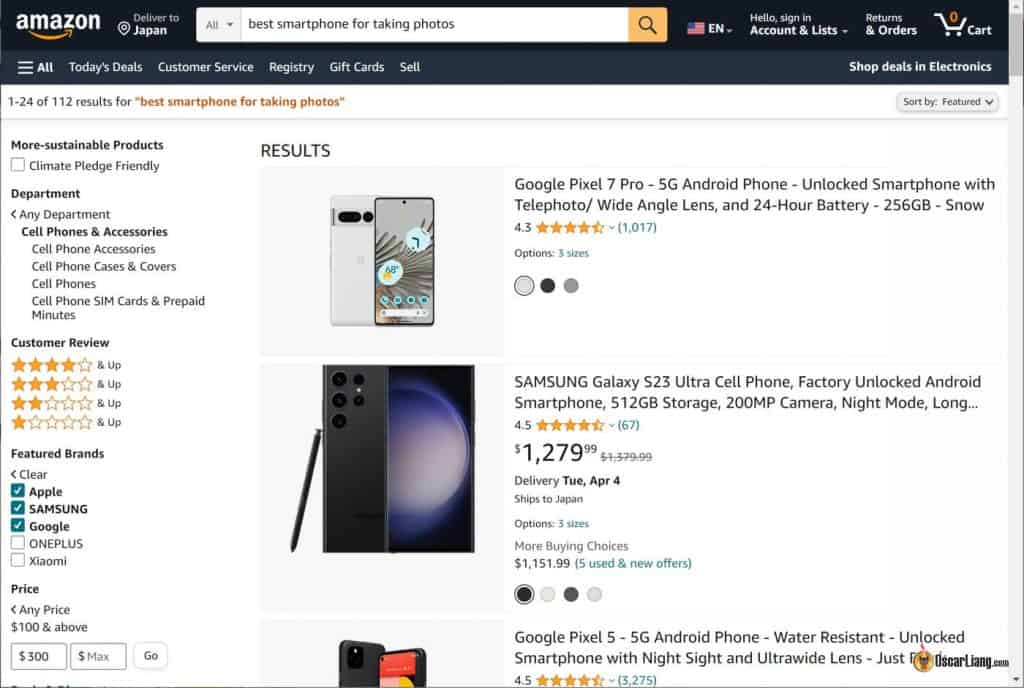The image displays the Amazon homepage, indicating an international user with the "Deliver to Japan" message situated next to the Amazon logo. The search bar contains the query, "best smartphone for taking photos," suggesting that a user from Japan is seeking recommendations for photography-oriented smartphones. This raises an interesting point about the use of Amazon as a platform for obtaining product advice, despite its primary function as an online retailer. This approach may result in biased suggestions driven by sales incentives, rather than unbiased advice typically found on review-focused websites.